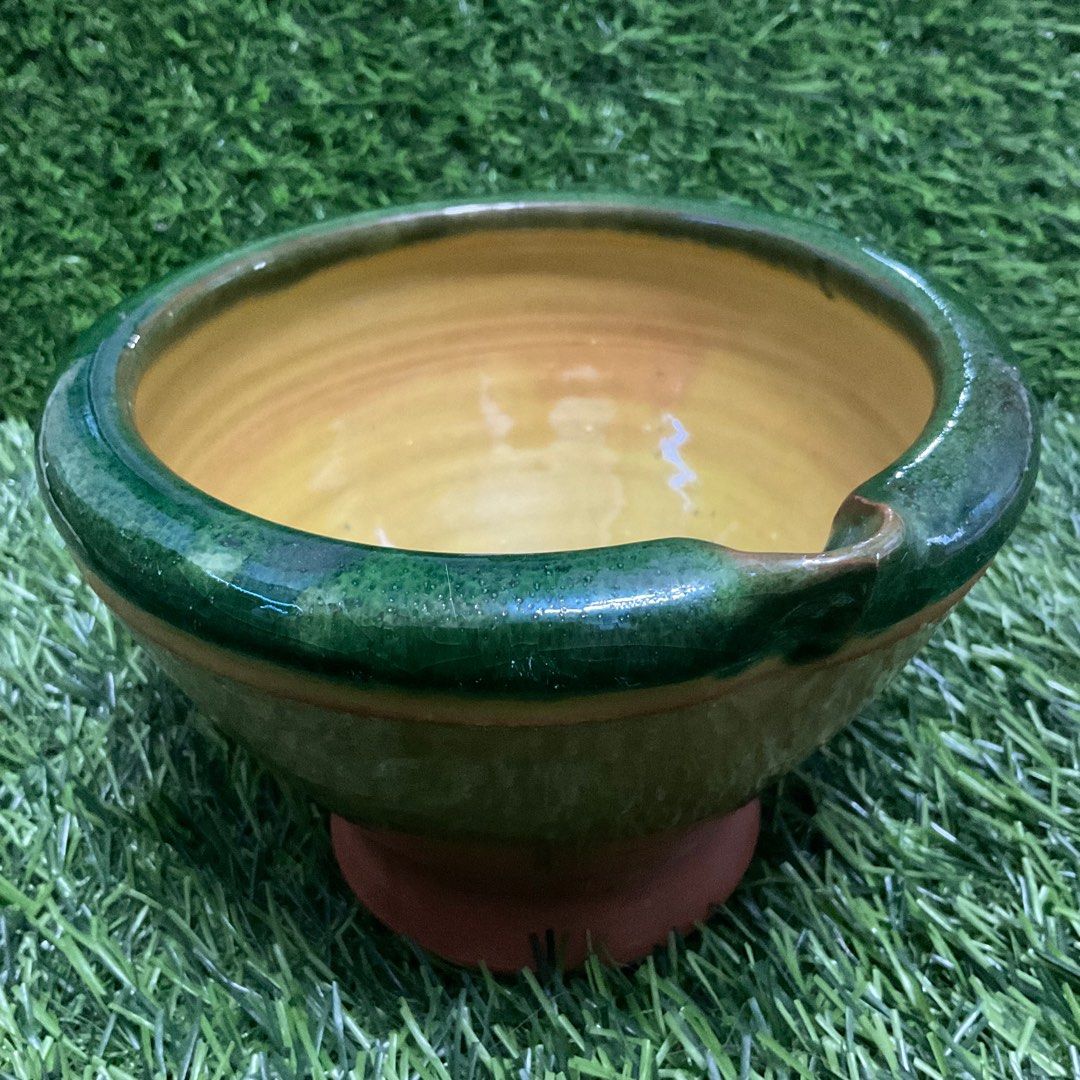The image captures a close-up view of a ceramic pottery bowl resting on meticulously manicured artificial green grass. The bowl's exterior features a dark green color with subtle variations and darker speckles, giving it a textured appearance. The base of the bowl is terracotta-colored, providing a sturdy foundation. It boasts a distinctly yellow, glossy interior and includes a small, spout-like indent on one side, likely designed for pouring. The photograph conveys a realistic and highly detailed visual, with shadows beneath the bowl enhancing its dimensionality.